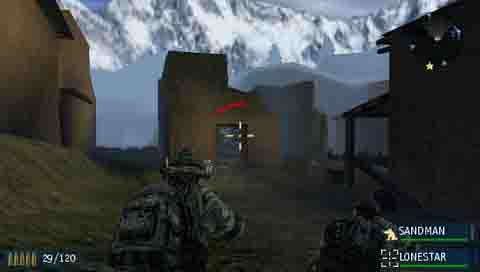In this detailed screenshot of a video game, we observe a combat-themed scenario set in an outdoor environment featuring several industrial-looking, rust-colored buildings. Prominently, a house in the center is marked with a target symbol and a red line above it. To the right of this house, another building hosts a distinctive yellow star, while a third building remains untouched. In the foreground, we see characters dressed in army fatigues and backpacks, walking toward the central target; their numbers are a bit hard to decipher, but it appears there are at least two, possibly three soldiers. The landscape behind these structures is dominated by huge, snow-capped mountains, indicating a cold climate setting. On the screen, in the lower-left corner, there is a display of ammunition, showing "29/120" bullets remaining. Additionally, the names "Sandman" and "Lone Star" are visible, likely identifying the players or characters involved in the game.